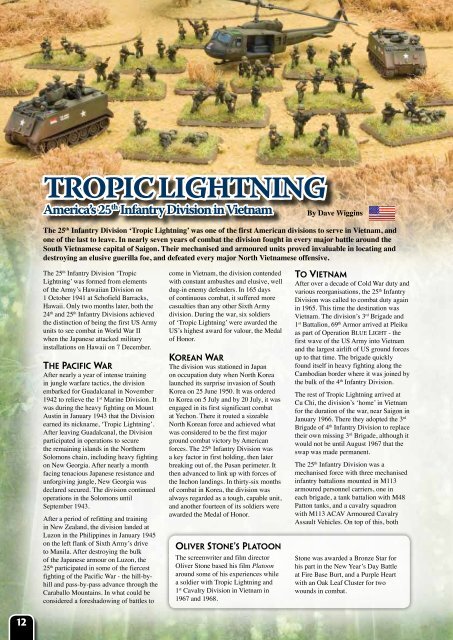This page from a magazine features an illustration depicting the 25th Infantry Division, known as Tropic Lightning, in Vietnam. The scene portrays soldiers, tanks, and helicopters set against a stark desert backdrop, with each element placed on separate grassy platforms, evoking the look of toy army men. The header, "Tropic Lightning: America's 25th Infantry Division in Vietnam," is prominently displayed in blue text, with the byline "By Dave Wiggins" and an American flag positioned to the right. The detailed article discusses the 25th Infantry Division, one of the first American divisions to serve in Vietnam and among the last to leave, highlighting its crucial role in major battles around Saigon over nearly seven years. Additional sections cover the division’s history, with the first paragraph referencing the Pacific War, followed by insights into the Korean War, and concluding with its involvement in Vietnam. There's also a mention of Oliver Stone's film "Platoon," with a brief description tying it to the division. The smaller resolution makes portions of the text challenging to read, but the rich visual and textual content vividly captures the storied legacy of Tropic Lightning.